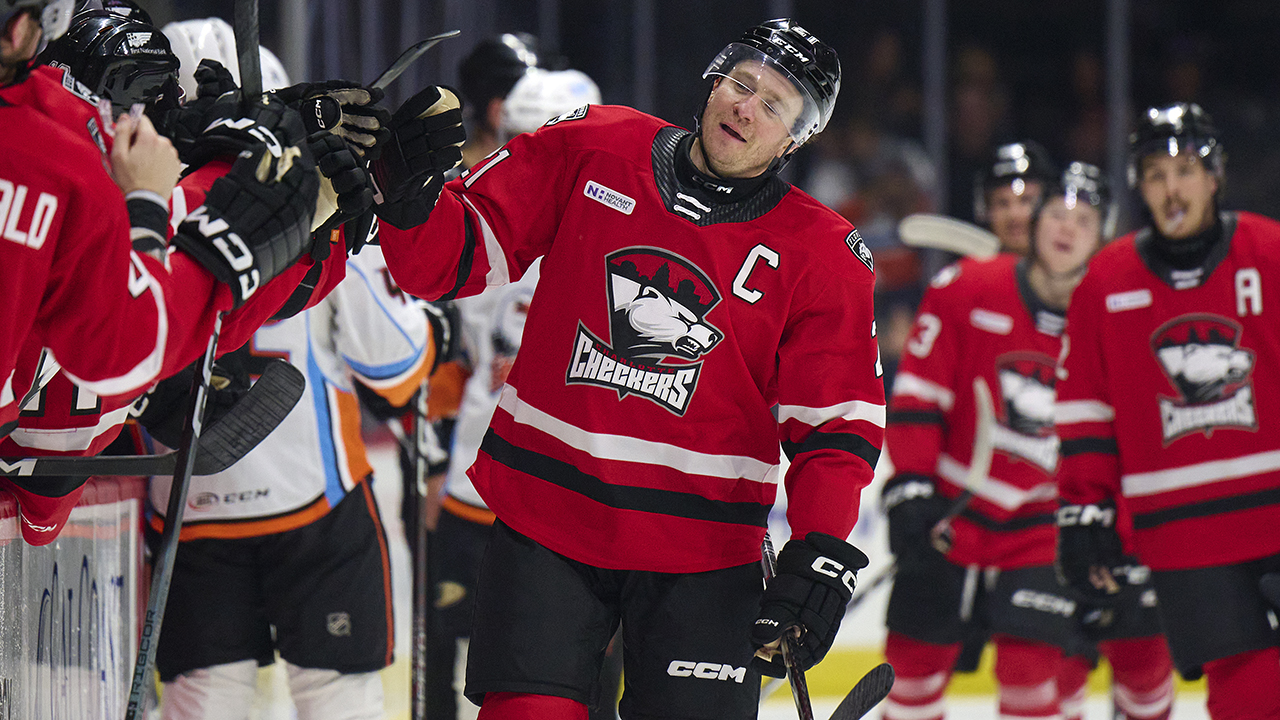In the image, we see the hockey team Checkers celebrating what appears to be a victory on an ice rink. The players are decked out in striking red, long-sleeved uniforms featuring a fierce white bear with a silhouetted red forest above it, and the word 'Checkers' below. The main focus is on the player at the center, wearing a black helmet and a white eye shield, distinguished by a large 'C' above his left chest, indicating his captaincy. He's smiling and doing a fist bump with another team member. The team members collectively wear black helmets, gloves, and shorts. To the right, another player sports an 'A' on his uniform, signifying an alternate captain. In the background, slightly blurred, are players from the opposing team dressed in white shirts with blue and orange stripes and black shorts. The scene is lively with a few spectators visible behind protective glass, highlighting the joyous and spirited atmosphere in the rink.